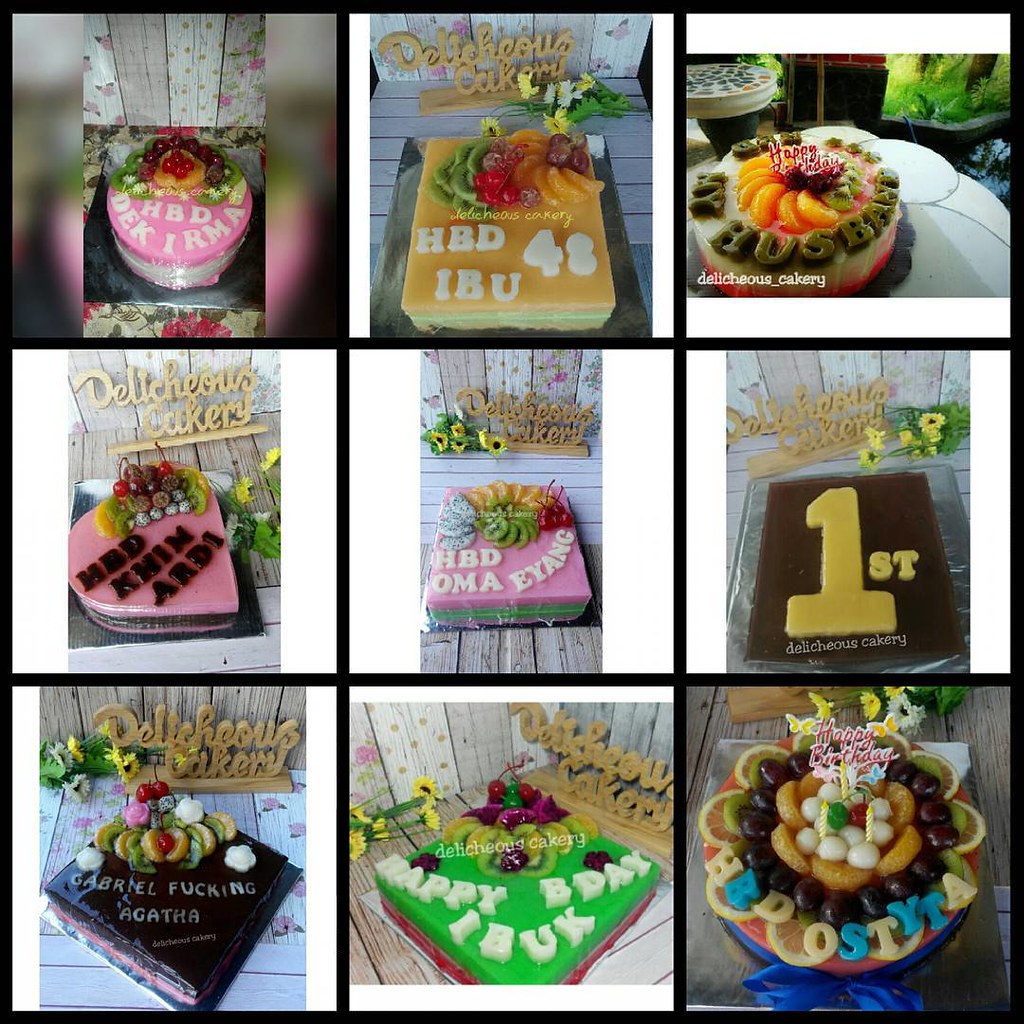This image features a 3x3 grid of nine photographs, each displaying different cakes from "Delicheous Cakery." Each square in the grid is bordered by a consistently thin black border, with no thicker outer border. The cakes showcase a variety of designs and messages, indicative of the bakery's custom capabilities. Here's a detailed caption for the image:

A grid of nine different custom cakes from "Delicheous Cakery," each with unique decorations and messages. The top left cake is pink with fruit and the text "HBD Dek Erma." Next is a yellowish sheet cake with the message "HBD IBU 48," adorned with fruit. The top right cake, a round one with peaches and kiwis, says "Happy Birthday" with the green text "My Husband." The center left cake is heart-shaped and pink, decorated with fruits, labeled "Delicheous Cakery." In the very center is another pink cake with white lettering "HBD Irma" and fruit. To its right is a chocolate cake with yellow lettering "First" and a large number one, suggesting it's a first birthday cake. The bottom left features a dark brown cake with white text "Gabrielle Agatha" and fruit toppings. In the middle bottom is a bright green cake saying "Happy B-Day IB UK," also decorated with fruit. The bottom right displays a round cake with orange, kiwi, and other fruits, labeled "Happy Birthday HBD OST YTA."